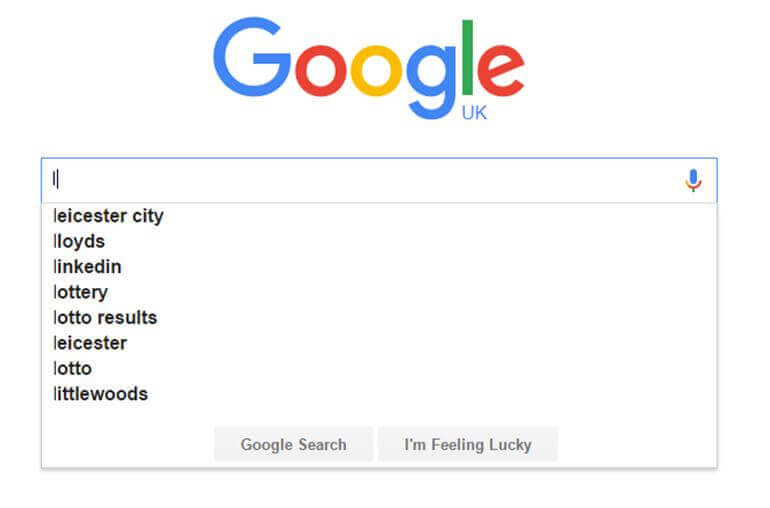A screenshot captured from Google UK showcases the iconic Google search interface against a clean, white background that seamlessly merges with the surrounding space. At the top, the vibrant Google logo is prominently displayed, featuring the signature color scheme: a blue 'G', red 'O', yellow 'O', another blue 'G', green 'L', and red 'E'. Just beneath the green 'L', the text 'UK' in small blue letters indicates that this is the UK version of Google.

Below the logo, the familiar search bar is present, complete with a microphone icon in the upper right-hand corner, signifying voice search capabilities. In the search box, an individual has initiated a query by typing the letter 'L'. Google's autocomplete feature has generated a list of suggested searches, including "Leicester City," "Lloyd’s," "LinkedIn," "Lottery," "Lotto Results," "Leicester," "Lotto," and "Littlewoods."

At the bottom of the screenshot, two grey rectangular buttons are visible, labelled "Google Search" on the left and "I'm Feeling Lucky" on the right. The format of the image, lacking any additional context or apparent device framing, leaves it ambiguous whether the interface is displayed on a mobile device or computer screen. However, it clearly depicts an initial search action on Google UK, with just the first letter typed in.